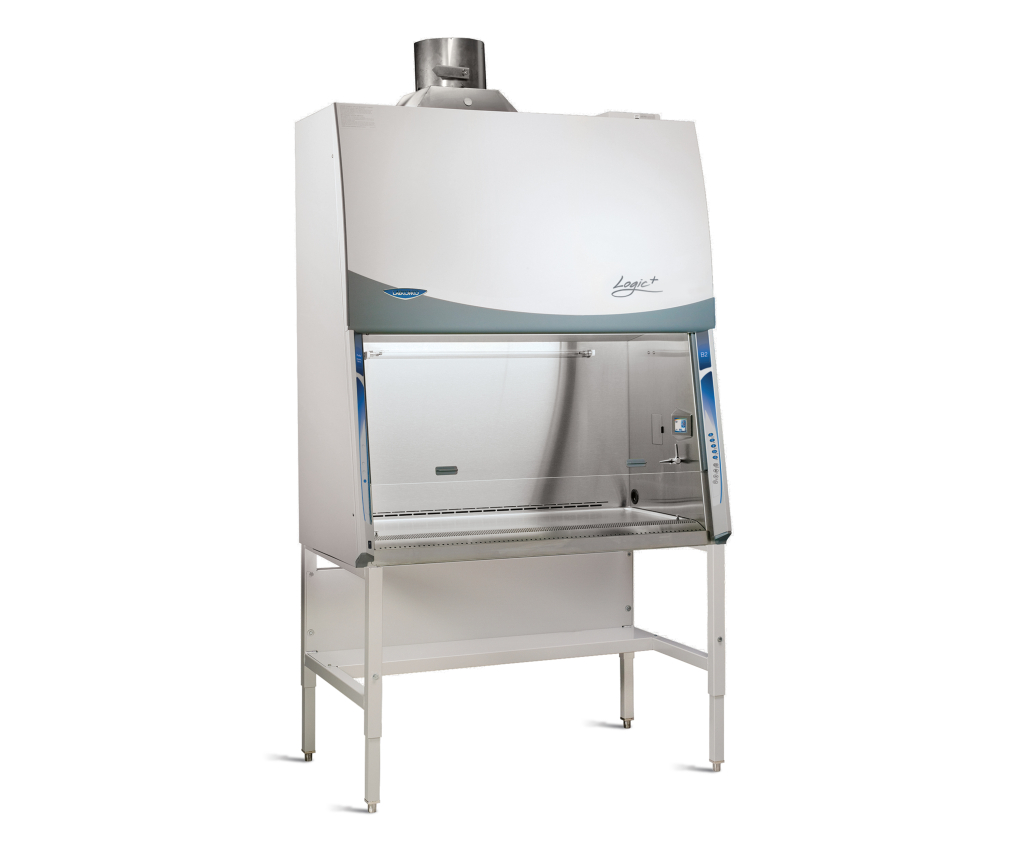The image depicts an intriguing and presumably specialized machine, possibly used in a medical or laboratory setting. The structure features a large metal frame made of either white or silver material, possibly blending elements of both. At the front of the machine, a glass pane reveals an interior compartment, suggesting the presence of a small door or shelf that can be opened to place items inside. This compartment appears to be illuminated and may include a grilling rack-like surface at the bottom. The machine rests upon four sturdy white legs. At the top, there is a cylindrical tube or metal gray exhaust, hinting at a function that involves either emitting or filtering air or gases. The machine is marked with the words "Logic Plus" in a distinctive swirly font, accompanied by a blue logo with unreadable writing. The overall design is sleek and modern, lending an air of sophistication and advanced utility to the device.